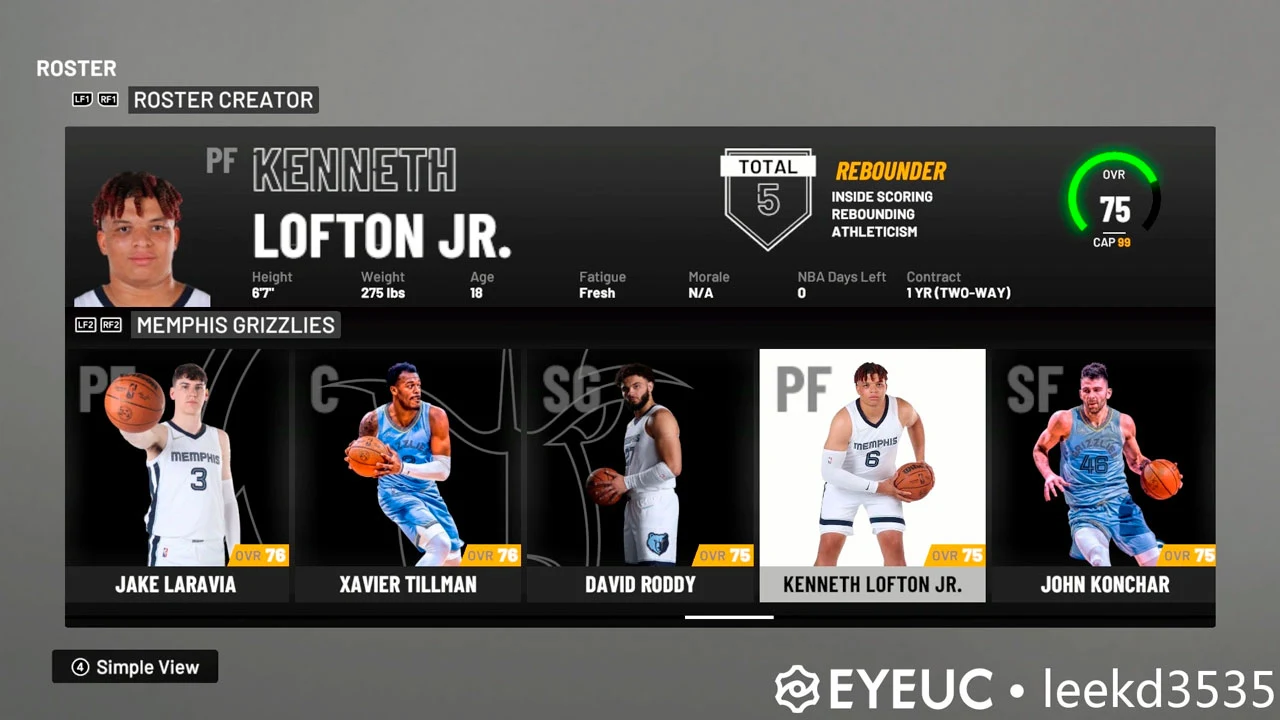This screenshot showcases a roster creator page prominently featuring basketball player Kenneth Lofton Jr. Standing 6'7" tall and weighing 275 pounds, the 18-year-old Lofton Jr. appears on the top banner, indicating he is the focal point. His status reads "fatigue: fresh" and "morale: N.A.," with details of his one-year two-way contract. Below his profile, the Memphis Grizzlies affiliation is clearly indicated, with five players listed beneath: Jake Laravia, Xavier Tillman, David Roddy, Kenneth Lofton Jr. again for emphasis, and John Conchar. A simple view button is located on the lower left side of the screen. On the lower right, a text displays the sequence "E-Y-E-U-C-L-E-E-K-D-3-5-3-5." The banner's background is black, adorned with faint watermarks reading "P-F-C-S-G-P-F-S-F."